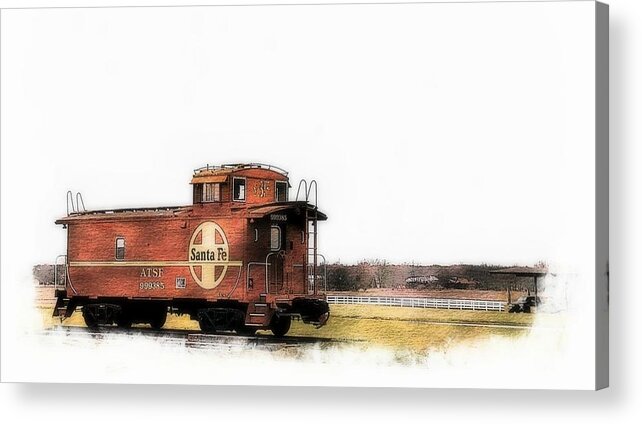The illustration depicts a stand-alone, vintage train engine set against a predominantly white background, likely rendered on a rectangular canvas or wood panel with a gray edge visible on the right side. The brown engine, adorned with a circular gold logo centered by a yellow cross and the text "Santa Fe," sits prominently on a set of tracks. Additional text, "ATSF," accompanied by a number, further details the engine. Its black wheels and front ladder contribute to the intricate design. To the right, a white picket fence runs parallel to a field of green grass tinged with yellow hues, extending towards a short, shrub-dotted brown hill. A platform-like structure with a roof stands near the fence, adding to the scenic transport setting. The bottom edge of the image appears cloud-like, blending into the background.